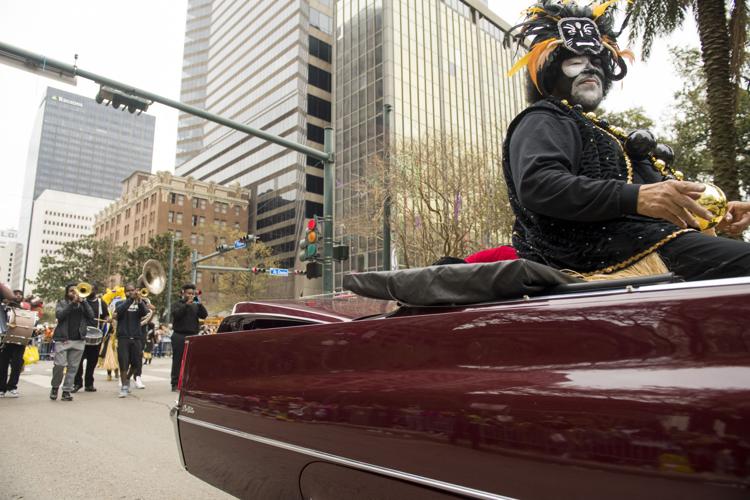The image depicts a vibrant Mardi Gras parade, captured from a low-angle perspective right next to a lengthy red Cadillac convertible with its top down. Seated prominently in the back of the car is a man adorned in an elaborate costume. His outfit features a black frilly coat with gold trim and black trousers. His face is painted with bold, theatrical makeup, including white spots around his eyes, a black nose, and black designs on his cheeks. Topping off his elaborate look is a dramatic headdress adorned with a black and white angry face, accented by colorful feathers in shades of black, green, yellow, and orange. Large beads are draped around his neck, signifying the festive Mardi Gras spirit.

Behind the convertible is a casual marching band consisting of African American youths dressed in street clothes, playing a variety of instruments such as trumpets, drums, trombones, and a tuba. The parade route is cordoned off, with towering office buildings, banks, and possibly apartment buildings forming the backdrop, interrupted occasionally by palm trees. This lively scene, filled with music and color, unmistakably captures the essence of a Mardi Gras celebration, likely in New Orleans.